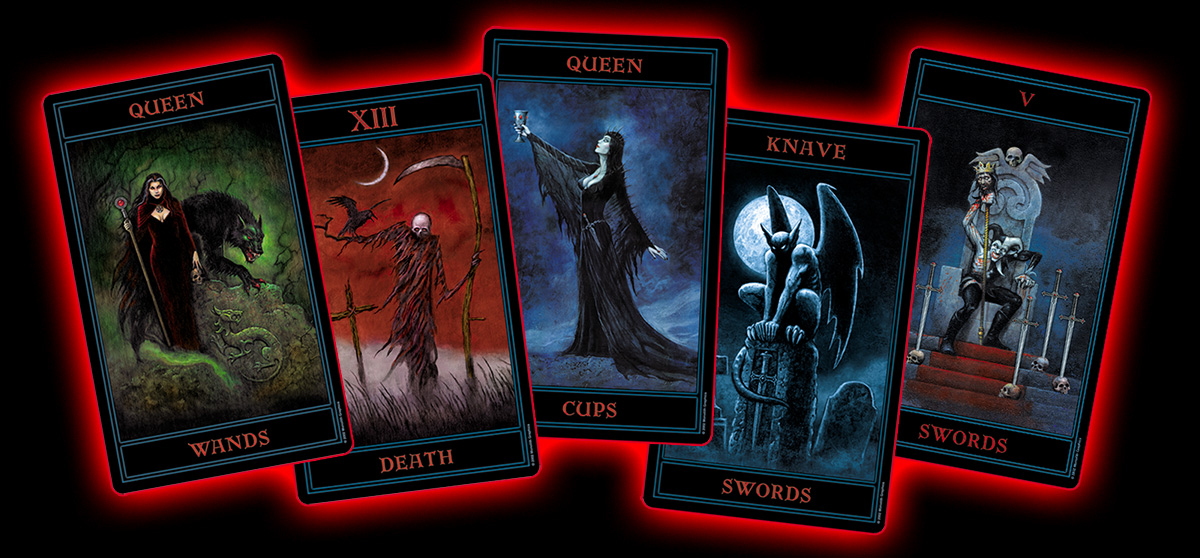The image features a collection of five intricately detailed, Gothic-themed tarot cards set against a stark black background. Each card is surrounded by a luminous red hue, enhancing their eerie aesthetic. The first card, titled "Queen of Wands," depicts a woman holding a staff, accompanied by a fearsome wolf. The second card, marked with the Roman numeral XIII (13) and named "Death," showcases a menacing skeleton wielding a scythe. The third card, labeled "Queen of Cups," features a Morticia Addams-esque figure in a long black dress, holding a cup. The fourth card, called "Knave of Swords," displays a gargoyle against a backdrop of a full moon. The final card, "V of Swords," presents a gruesome scene with a jester seated on a king’s chair, brandishing a sword impaling a royal head, surrounded by skulls with swords through them. Each character is vividly animated, contributing to the modern, darkly gothic ambiance of the deck, with all text and numerals highlighted in striking red.